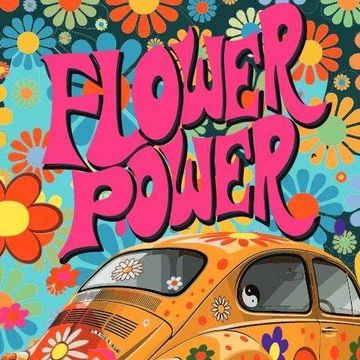The image depicts a vibrant and colorful piece of artwork, reminiscent of a 1960s psychedelic poster, featuring bold graffiti elements. At the bottom right corner, there is an orange Volkswagen adorned with an array of flowers and symbols, including daisies and a yin-yang on one of the windows. The car is elaborately decorated with flower decals in various colors, adding to the overall vividness. The background consists of a wall covered with mod-colored daisies in shades of blue, orange, gray, yellow, pink, purple, lavender, and green, creating a diverse and lively atmosphere. Centrally positioned towards the top of the image, the text "Flower Power" is written in a fancy, bold pink font, emphasizing the 70s style. This artistic piece showcases a captivating blend of retro aesthetics and modern graffiti art, with a rich palette of colors enhancing its visual appeal.